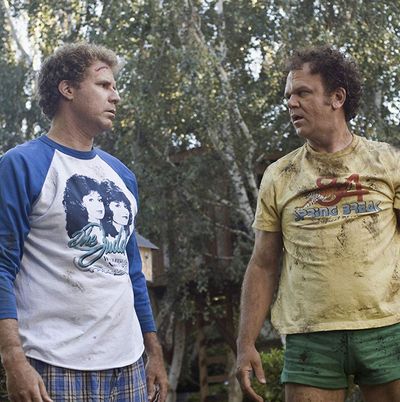In the image from the movie *Step Brothers*, both brothers, played by Will Ferrell and John C. Reilly, are intensely facing each other with expressions of anger and confusion, clearly having just gotten into a fight. Dirt marks are splattered across John C. Reilly's yellow "Prime Breck 84" t-shirt, and Will Ferrell has a visible cut on his forehead. Ferrell is dressed in a distinctive blue and white baseball tee adorned with the Judd sisters’ image, with its sleeves rolled up, paired with checkered plaid pants. John C. Reilly sports green camouflage short shorts. Both men have curly hair and stand amidst a backdrop of dense trees, through which some sunlight and patches of pale blue sky are visible, adding a serene contrast to their disheveled appearances.